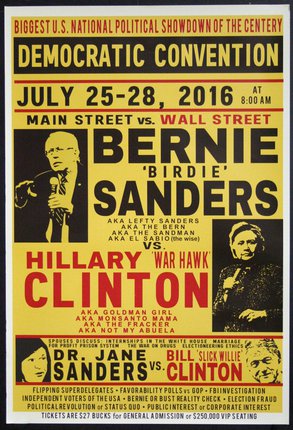This image is a scanned political poster from 2016, characterized by its black border and primarily yellow background. At the top, the poster dramatically announces "Biggest U.S. National Political Showdown of the Century," though it misspells "century" as "centery" in red letters. Below, it promotes the "Democratic Convention" from July 25th to 28th, 2016, at 8 a.m., highlighting the clash as "Main Street versus Wall Street."

The central figure of Bernie Sanders is depicted with multiple nicknames: "Birdie Sanders," "Lefty Sanders," "The Bern," "The Sandman," and "El Sabio, The Wise." His opponent, Hillary Clinton, is labeled with disparaging monikers: "Warthog Clinton," "Goldman Girl," "Monsanto Mama," "The Fracker," and "Not My Abuela." This framing strongly suggests the poster was created by Bernie Sanders’ supporters or someone antagonistic towards Hillary Clinton, likely emphasizing Sanders as the candidate of the people (Main Street) versus Clinton as the candidate of corporate interests (Wall Street).

The poster also humorously pits Dr. Jane Sanders against Bill "Slick Willie" Clinton, accompanied by cartoonish representations of both individuals. At the very bottom, it touches on the public's interest in corporate influence and GOP favorability polls. Ticket prices are listed as $27 for general admission and an exaggerated $250,000 for VIP seating. The overall tone and presentation imply a potentially far-right or sharply critical perspective on the Democratic primary candidates.